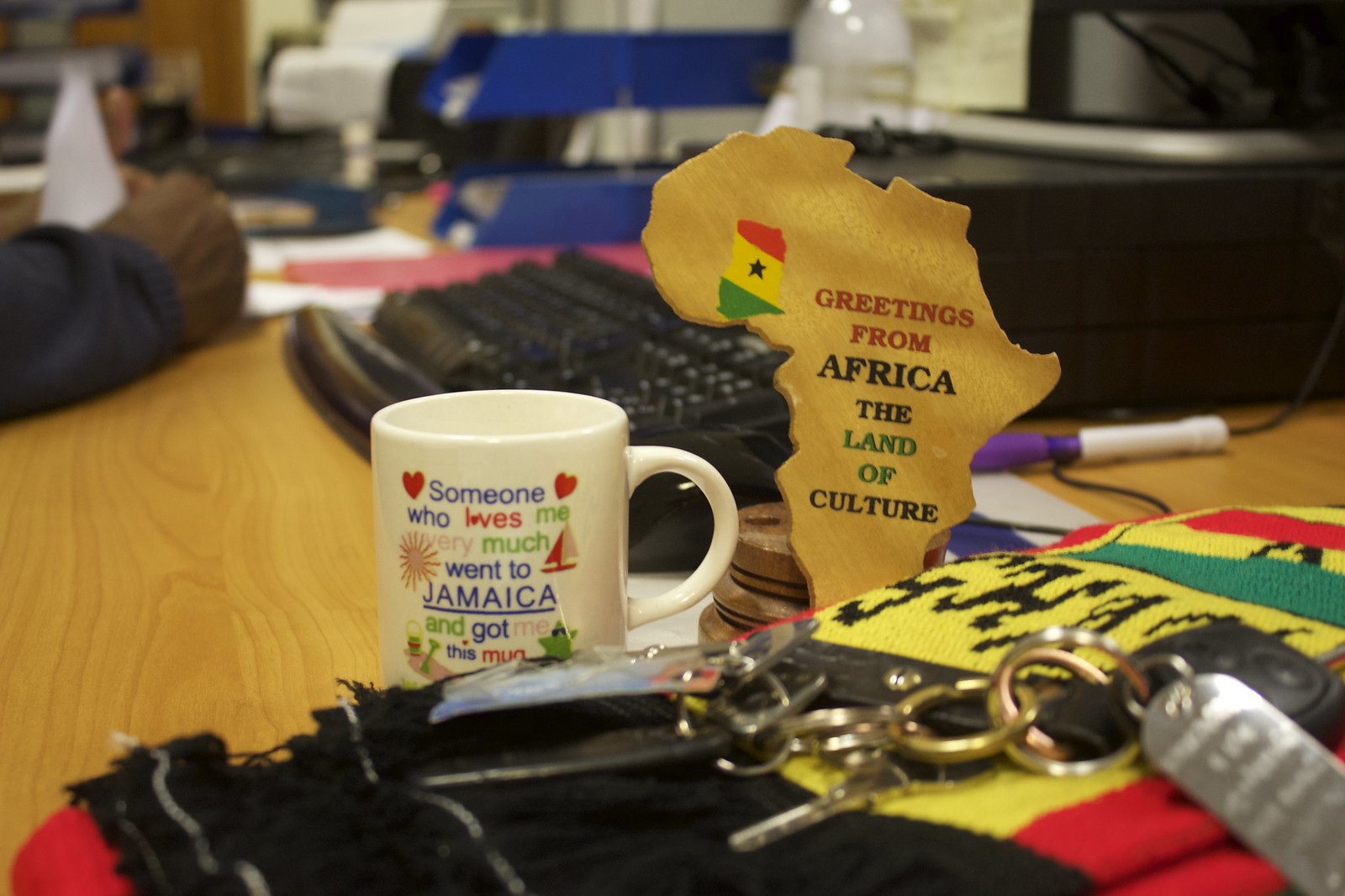The image captures a detailed view of a workstation, highlighting both personal and cultural items. At the forefront, on a colorful blanket woven with black, yellow, red, and green stripes, lies a set of card keys. Partially covering the blanket is a white coffee mug adorned with mixed blue, red, and green text that reads, "Someone who loves me very much went to Jamaica and got me this mug." The mug also features a sun silhouette and a sailboat, although partially obscured by the blanket.

Adjacent to the mug, there's a brown wooden cutout of Africa, positioned next to a flag that is red, yellow, and green with a black star at its center. The flag appears slightly torn. Inscribed near the flag, the text reads, "Greetings from Africa, the land of culture," with the words "Greetings from" in red, "Africa," and "culture" in black, and "land of" in green.

In the background, a black keyboard and the base of a desktop computer are visible, the latter partially hidden behind the African cutout. To the left, a person's hand, seemingly belonging to a black individual wearing a dark blue jacket or long-sleeved shirt, is visible. Additional items in the blurry background include white and pink papers and possibly a printer with paper coming out of it.

Overall, the image intricately combines elements of everyday work life with items reflecting cultural pride and personal connections.